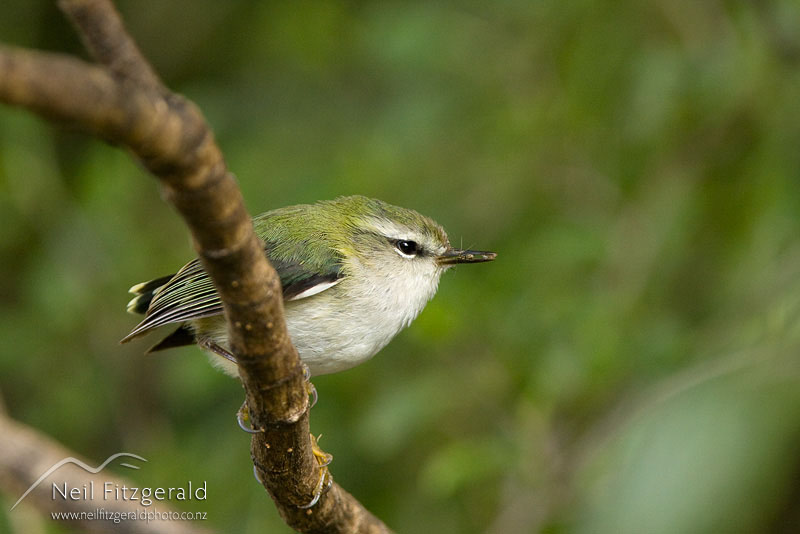This high-resolution wildlife photograph captures an exquisitely detailed, small chubby bird perched on a narrow, brown tree branch against a softly blurred green background. The bird, possibly a kinglet, showcases a vibrant mix of colors; its upper parts are adorned with greenish-yellow feathers that blend seamlessly into the natural surroundings, while its underbelly is white. The wings feature a distinct black and white pattern, with a noticeable black tail tipped with light green or white feathers. The bird's slender, dark beak and small, black eyes are punctuated by a subtle white eye ring and a black eye stripe. Additional whisker-like fibers extend around its beak. Its feet, with impressively large claws, grip the branch securely. The image also contains a watermark in the bottom left corner, reading "Neal Fitzgerald" alongside a stylized mountain logo and the website "www.nealfitzgeraldphoto.co.nz," indicating the photographer's New Zealand origin. This photograph beautifully highlights the bird's vivid detail against a lush, out-of-focus backdrop, presumably a dense green forest or shrubbery.